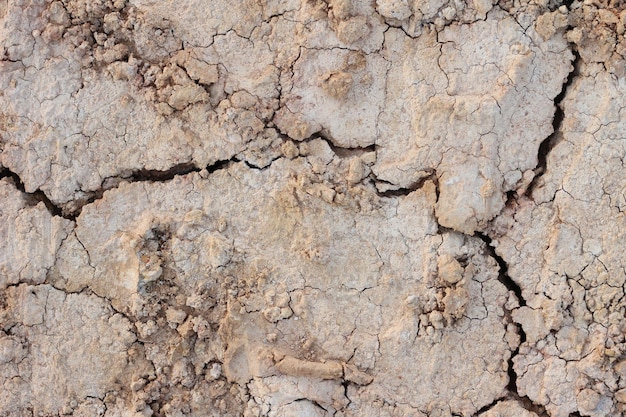This close-up aerial photographic image, likely taken by a drone, captures an outdoor scene featuring a parched, barren expanse of dry soil. The ground is primarily brown with flecks of orange, interspersed with prominent black fissures and veins that give the soil a cracked, crumbly appearance. One significant fissure extends from the left edge of the image, traversing diagonally across before bending downward and ending in the lower right-hand corner. Another prominent crack branches upward toward the top right corner. The soil appears extremely dry and in desperate need of moisture, highlighted by the light-colored cracks and the overall crumbly texture indicative of severe dryness and recent environmental changes.